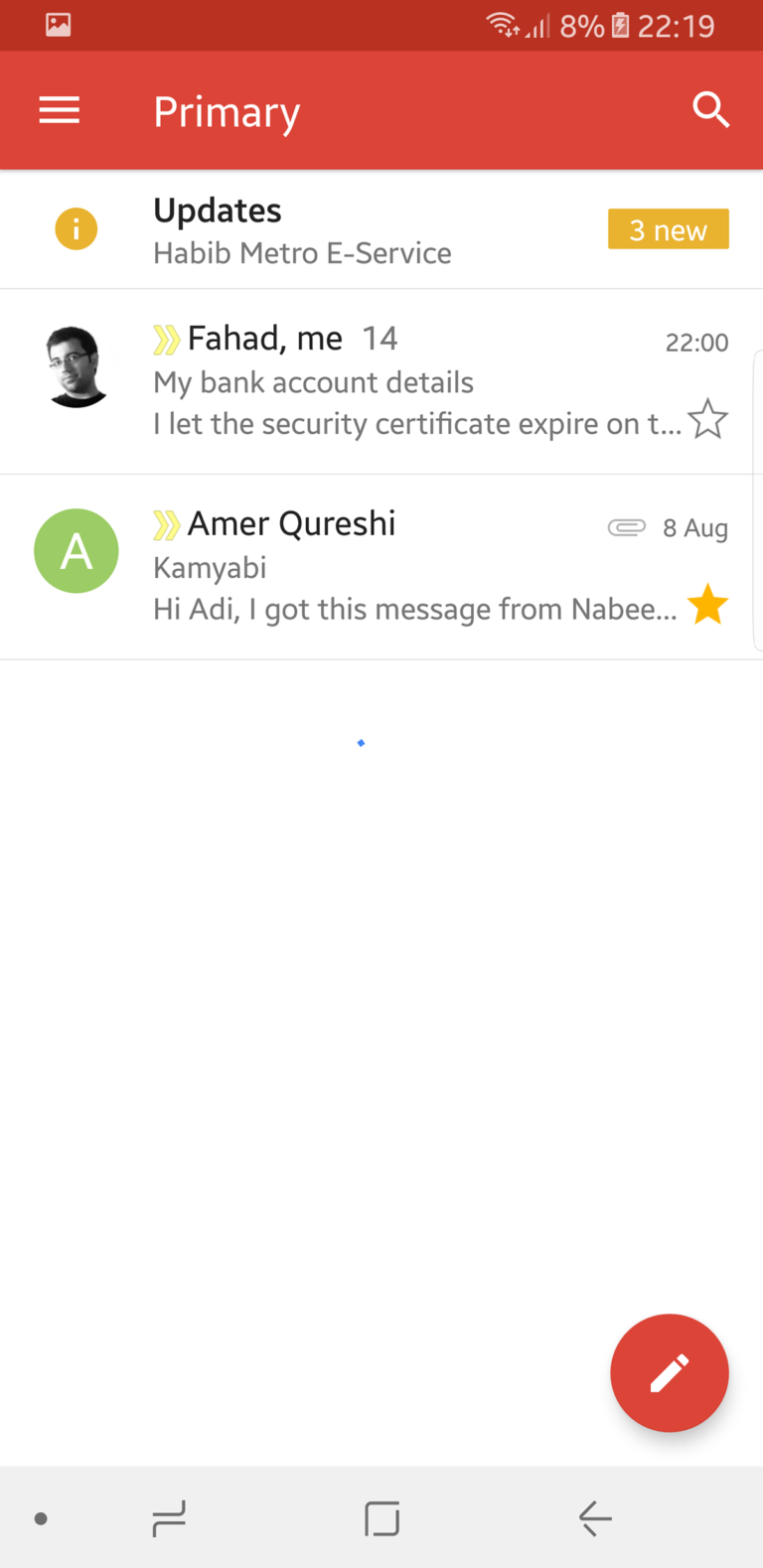Here is a cleaned-up and detailed caption for the image described:

---

The screen display of a device is divided into two distinct sections with a red background at the top and a white background at the bottom. In the upper-left corner, there is a picture icon. Adjacent to it on the right is a Wi-Fi icon, followed by a cellular signal icon. To the right of these icons, the battery percentage is displayed, reading "8%," accompanied by a battery icon indicating its charge status. Further right, the current time is shown as "22:19."

Just below this display area, on the left side, there's a "More" icon. To its right, the word "Primary" is spelled out ("P-R-I-M-A-R-Y"). On the far right is a white search icon.

In the bottom section of the screen, on the left, there is a yellow and white information icon, next to which the word "Updates" is written. Below this, it displays “Habib Metro E-Service” (spelled “H-A-B-I-B” Metro E-Service). Positioned on the far right are the words "3 new."

In the section beneath this information, there is an image of a man on the left side of the screen.

---

This version provides a comprehensive description and corrects any inconsistencies in the original text.